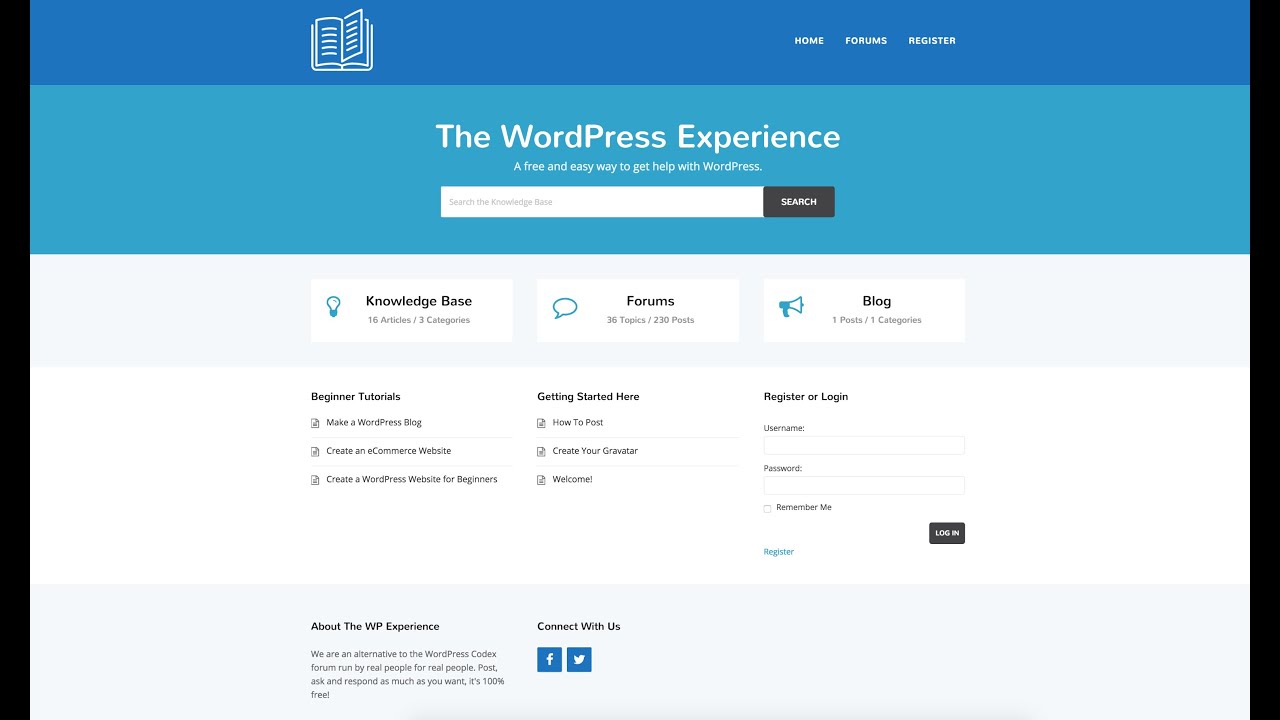The image depicts a comprehensive help page for WordPress users, designed to be a free and user-friendly resource for those seeking assistance with the platform. At the top, a prominently featured search bar allows users to easily locate specific information. Directly below, the page is organized into several distinct sections: Knowledge Base, Categories, Forums, and Blog. Each section provides targeted content, such as beginner tutorials and a "Getting Started" guide, to help users navigate WordPress.

Additionally, the help page includes options to register or log in, offering a more personalized support experience. A community chat area is also available, fostering a collaborative environment where users can ask questions, address concerns, and share tips on using WordPress effectively. Contact options are provided for further support via social media channels like Facebook and X (formerly Twitter).

Visually, the page features a gradient design, with a lighter blue header and a gray footer. Text is primarily black, ensuring readability against the background. The WordPress logo, displayed in white, adds a touch of branding to the help page, reinforcing its purpose as an official resource for users.